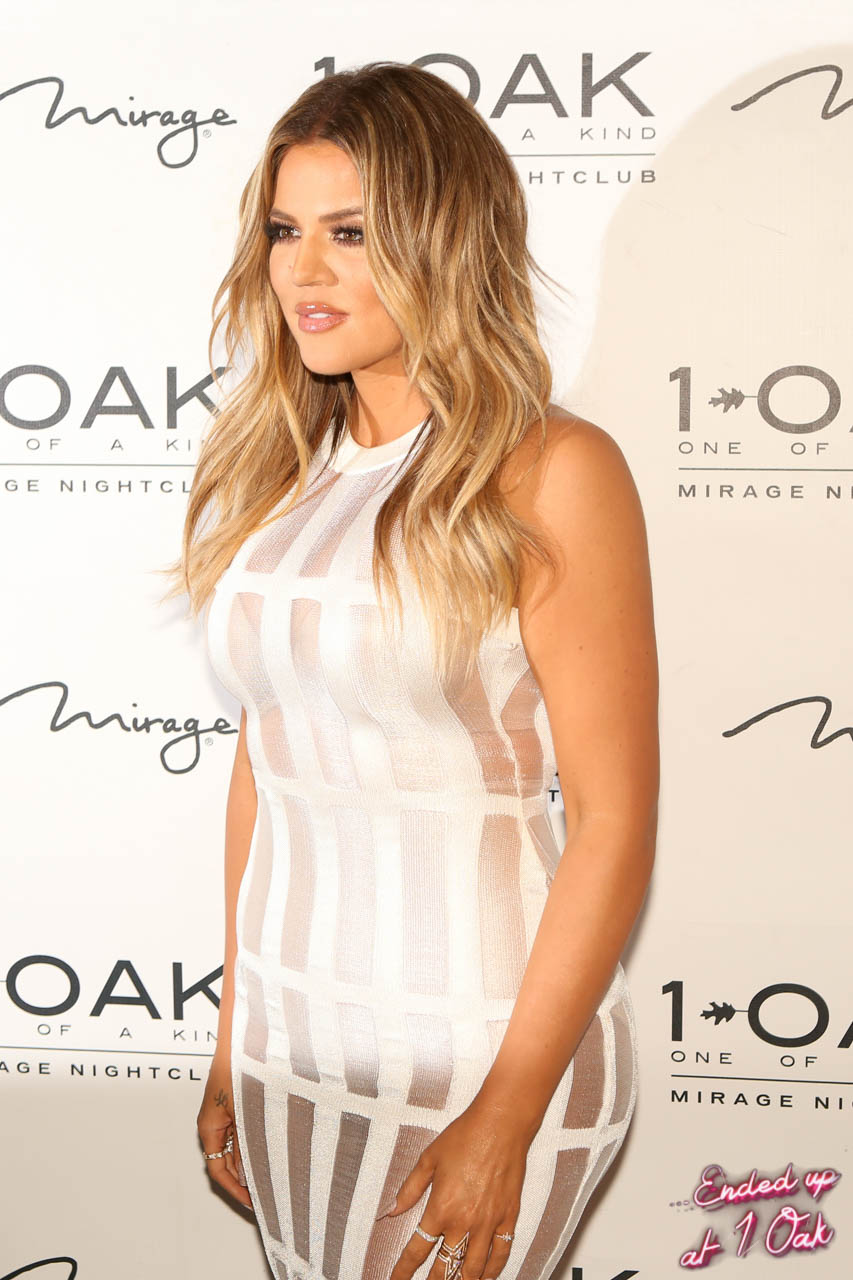The image captures a woman, strongly resembling Khloe Kardashian, standing confidently at a red carpet event in front of a white backdrop adorned with the repeated text "Mirage" and "One Oak," as well as phrases like "one-of-a-kind Mirage nightclub." The backdrop also features cursive white and pink lettering stating "Ended up at One Oak." The woman has light brown hair with blonde streaks cascading past her shoulders and is looking slightly to the left. She wears a stunning, form-fitting, sleeveless white dress with vertical and horizontal lines, featuring see-through material on the sides, and her attire adds a touch of shimmery silver. The dress is cut off just above her knees in the photo. Her makeup is natural, and she accessorizes with rings on every finger, as her arms rest by her sides. An evident light source from the left side casts her shadow to the right, enhancing the overall composition of the photograph.